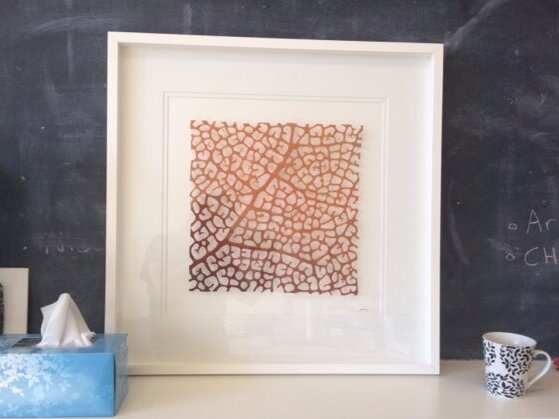The image is a detailed photograph showcasing a serene, carefully arranged scene. At the center is a square picture in a white frame, leaning against a chalkboard. The framed graphic within appears organic, featuring a flat, light orange background interwoven with light gray, vein-like patterns reminiscent of a tree or a kiata leaf. The chalkboard behind it is black, adorned with chalk smudges and partially erased lettering, adding a touch of casual authenticity. On the white table supporting the picture, a blue tissue box sits in the left bottom corner, while on the right side, a white mug with black floral designs stands, suggesting a moment of quiet reflection or creativity. Together, these elements create a harmonious and inviting atmosphere.